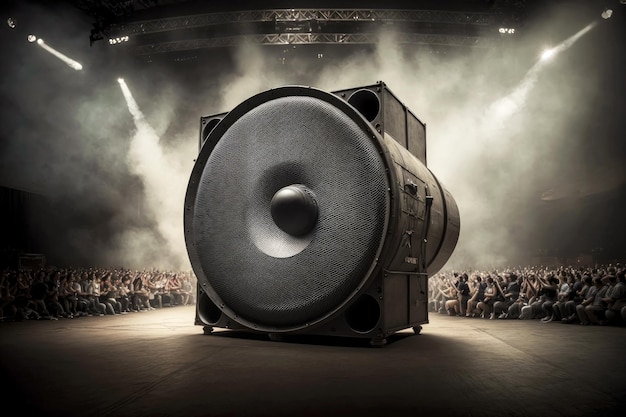The photograph depicts an enormous, surreal speaker positioned centrally within an auditorium or concert-like setting, radiating a dramatic spectacle. This monumental speaker, seemingly around 20 feet tall, is designed with a circular speaker component encased in a metal frame, accompanied by four large tweeters situated at each corner of the frame, each approximately two feet tall. The scene is enshrouded in smoke, adding to the dramatic ambiance, with lights from the rafters and possibly daylight filtering through, creating striking illumination on the speaker. The backdrop is filled with an enthusiastic crowd of possibly a hundred or more attendees, many of whom have their arms raised, some cheering, enhancing the sense of awe and excitement. The seating consists of folding chairs, reinforcing the temporary nature of the setting, akin to a gymnasium or an auditorium prepared for a significant and mesmerizing event. The image's overall composition and lighting suggest it could be a highly stylized 3D rendering or an artist's representation, adding an element of the surreal to the already extraordinary scene.